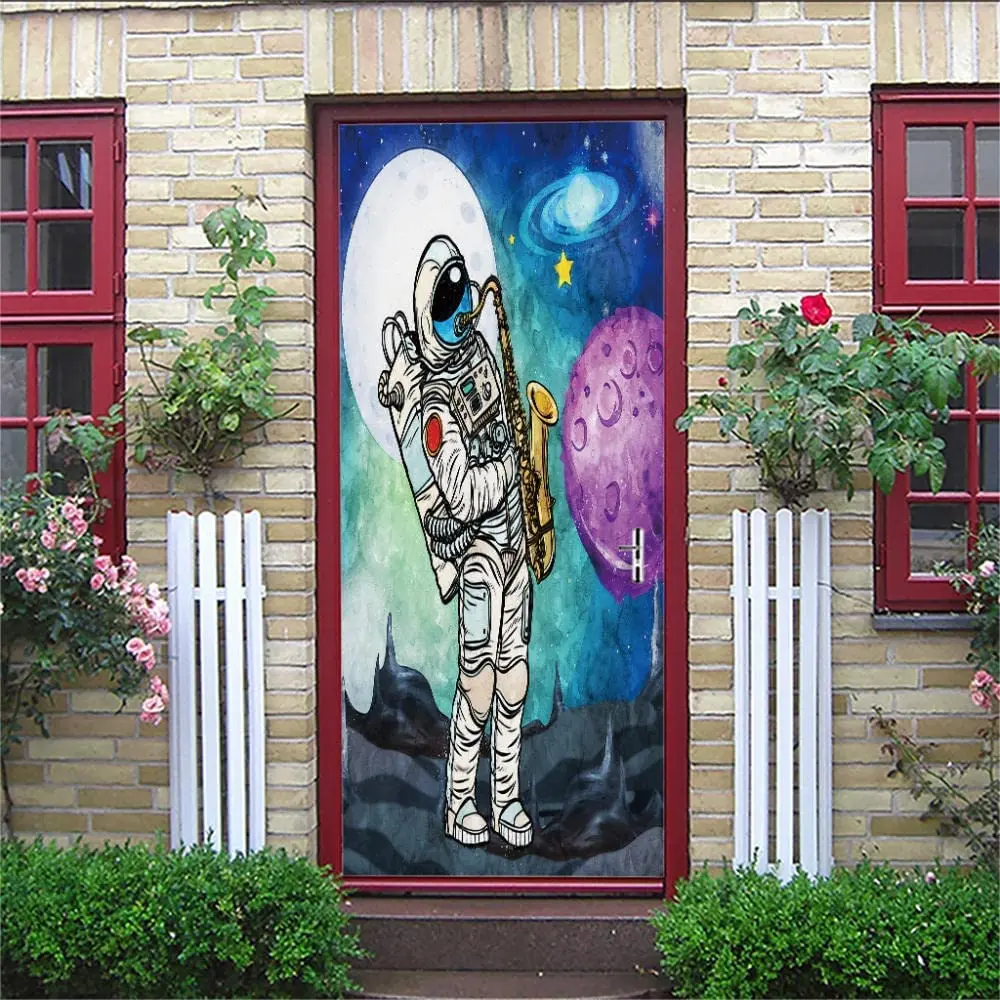This vibrant and photorealistic image captures the entrance to a well-maintained private home or apartment, surrounded by lush foliage and detailed greenery. The focal point of the scene is a front door adorned with an eye-catching mural depicting an astronaut in a full space suit, playing a saxophone. The astronaut stands against a dark gray, wavy surface, reminiscent of the moon's terrain. Behind the astronaut, a purple planet and another celestial body designed to resemble Jupiter add depth to the scene, along with scattered yellow stars in a detailed artwork. The windows on either side of the door are framed and painted in red, matching the door's outline, creating a cohesive and colorful aesthetic. Small green bushes and some flowering plants, possibly roses, add to the inviting atmosphere of this entrance, with circular fences outlining some of these plants. The overall scene appears to be photographed during the day, likely in the spring or summer, highlighting the home's attractive and glossy appearance.